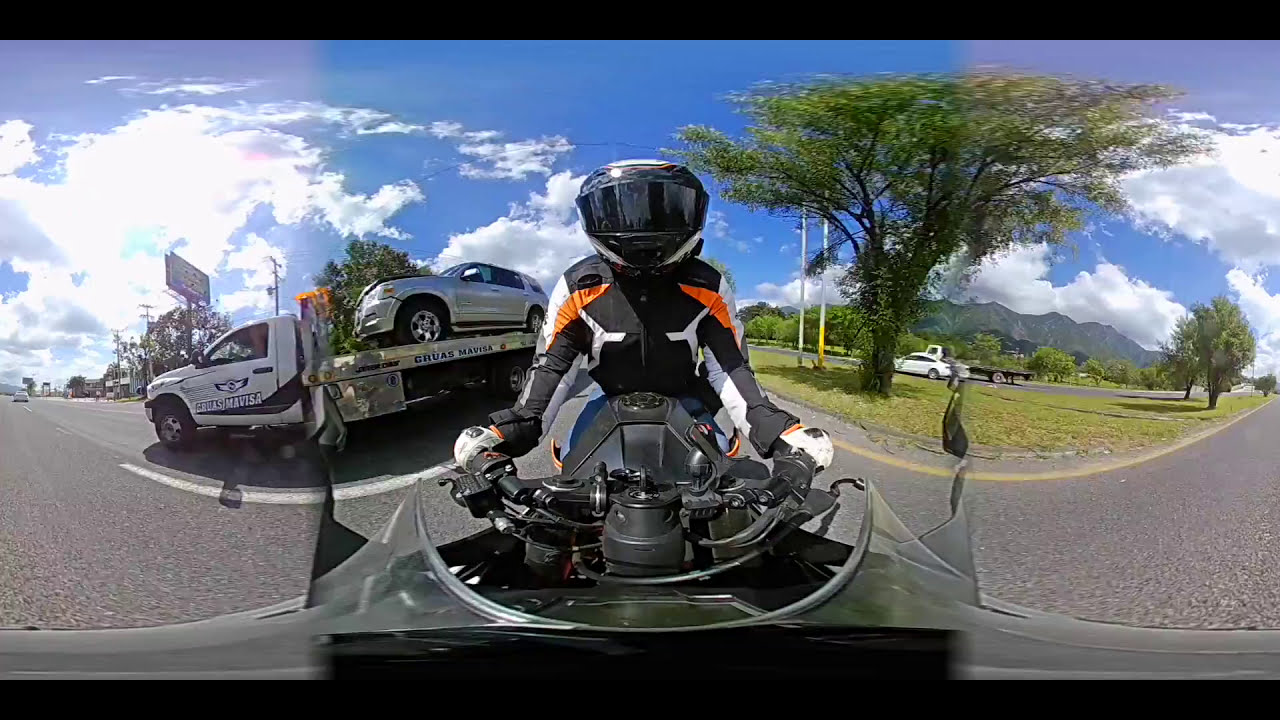This detailed image captures a person, likely female, positioned to drive a motorcycle. The rider is depicted in a dynamic stance, leaning slightly forward with hands gripping the handlebars. She is wearing a dark helmet with the visor down, obscuring her face, a predominantly black jacket accented with orange and white stripes, and white riding gloves featuring black accents. Her outfit is completed with blue jeans. The photograph appears to be taken from a rear-facing dash cam attached to the motorcycle, presenting a wide-angle view. 

In the background, on the left, there's a white tow truck carrying a silver SUV, situated in what seems to be a parking lot connected to a road. To the right, a tree with green leaves is visible, among other trees and a grassy median strip that divides the road. The setting is during daylight under a sunny blue sky dotted with clouds, complementing the scene's bright and vibrant atmosphere.